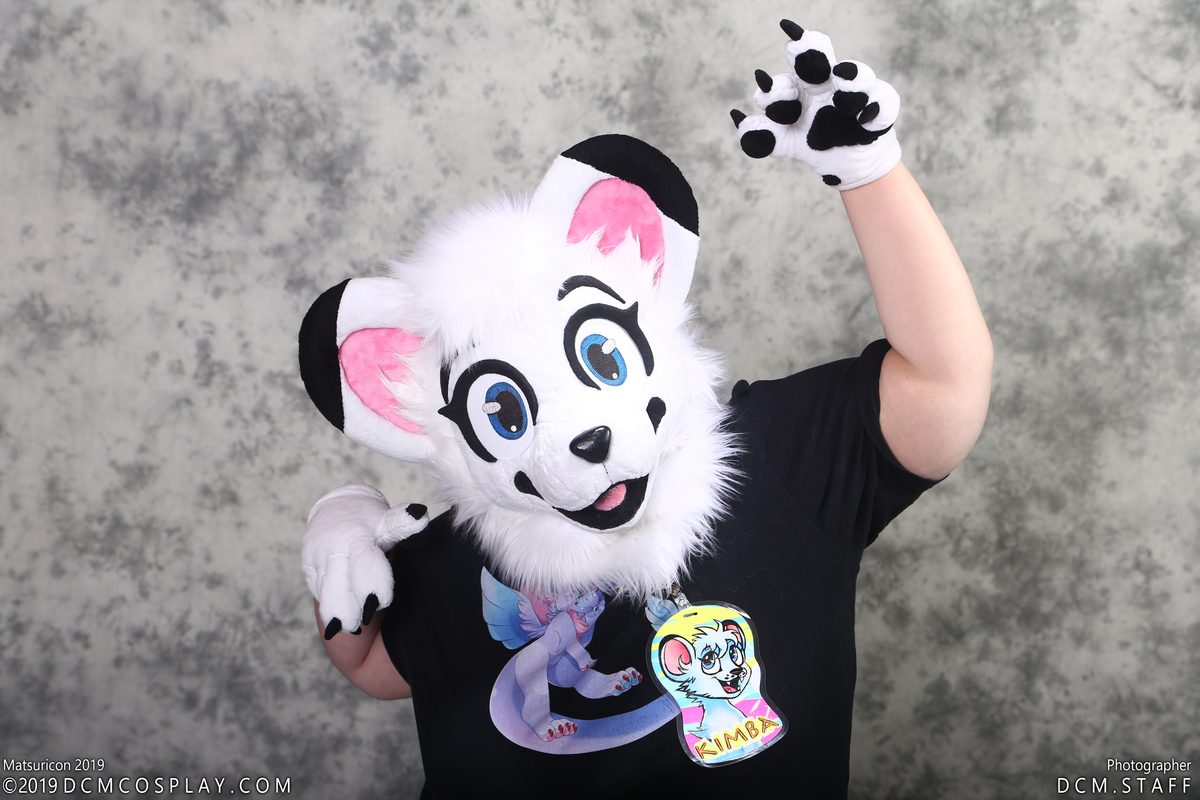This professional photograph captures a person cosplaying as a furry character named "Kimba." The individual is wearing a detailed, full-head mask depicting an anthropomorphic animal, most likely a white-colored fox, with expressive blue eyes, pink and black ears, and a smiling face. The outfit is completed with matching black and white gloves designed to resemble animal paws, featuring black claws and pads. They are also dressed in a black short-sleeved t-shirt that displays an image of the same character, Kimba, along with a name badge that reads "Kimba." The background consists of a gray, textured wall, characteristic of professional portrait settings. The photograph includes text at the bottom left corner stating "DCM Cosplay.com 2019" and at the bottom right corner, it reads "DCM Staff Photographer," indicating that the image was taken at a cosplay event by a professional photographer.